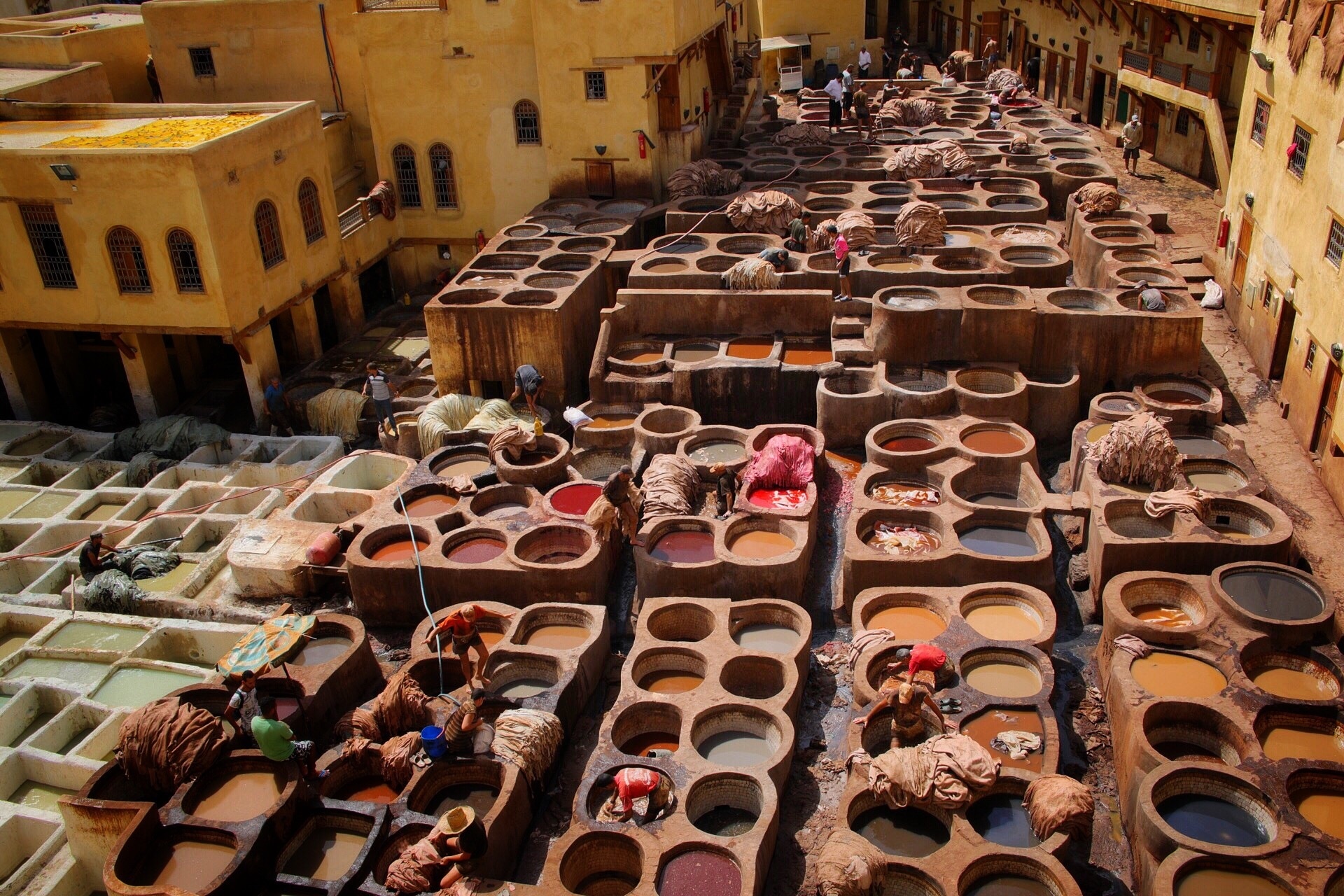This aerial photograph captures the bustling tannery of Fez, Morocco, renowned for its traditional leather dyeing process. Dominating the scene are rows of interconnected, tall vats or cauldrons filled with a vibrant array of colored dyes—from gray, yellow, and blue to purple, brown, pink, and red. These vats are arranged in extensive rows, each comprised of clusters of five or more, stretching from the bottom to the top of the image. Surrounding this intricate network of dye-filled vats, several workers are seen navigating and tending to the materials, underscoring the depth and size of these structures. Draped fabrics hang from many of the vats, further illustrating the dyeing process in action. Framing this industrial tableau, old buildings with distinctive arched windows—some painted yellow and others a sandy hue—flank the left and right sides of the image, providing a striking contrast to the vivid colors below and completing the vivid, historical tapestry of Fez’s traditional tannery.